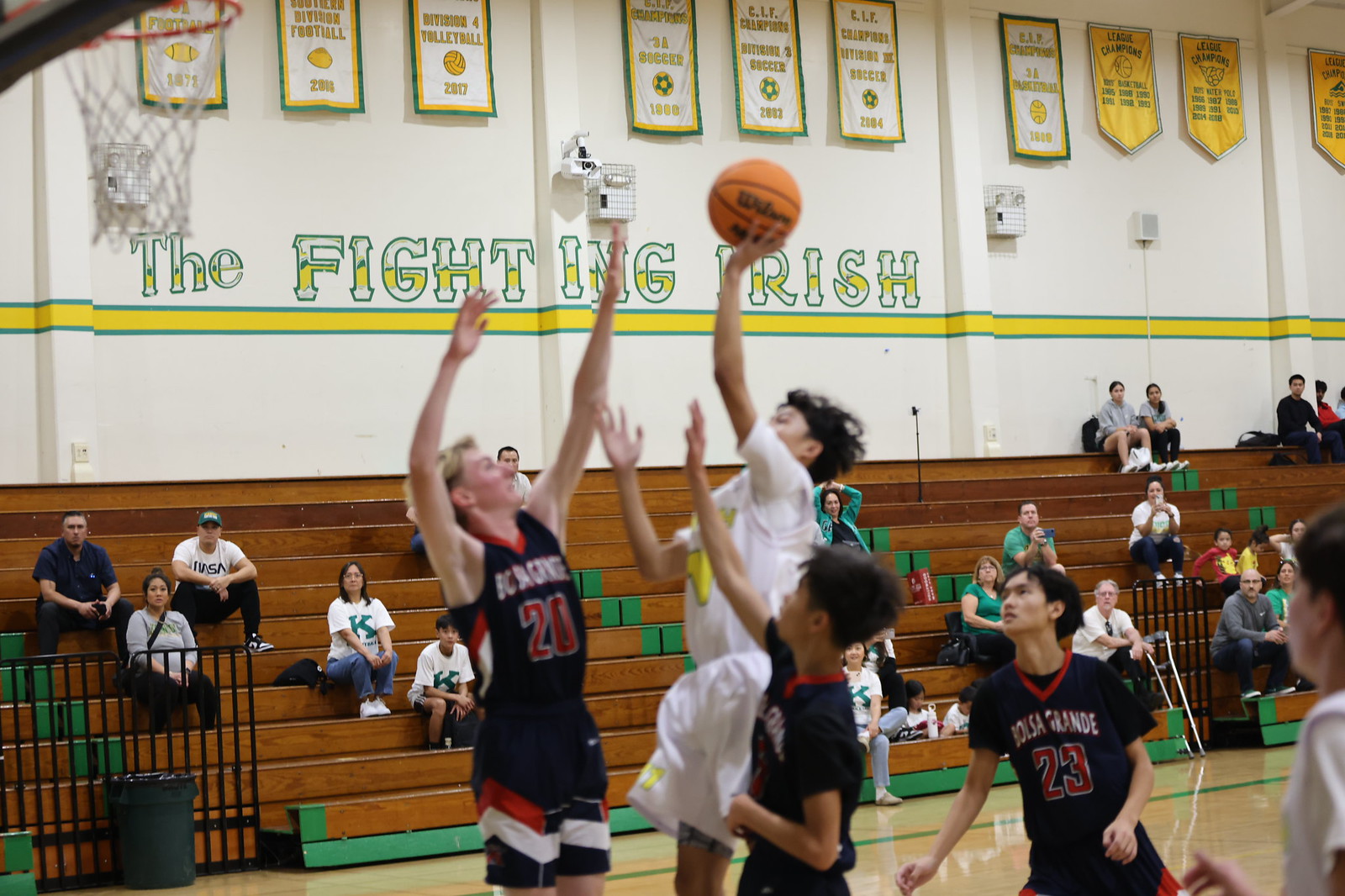The photograph captures an indoor high school gymnasium during a basketball game. It is about six inches wide and four inches tall. The scene is lively with two teams of high schoolers on the court; one team wears black and red uniforms while the other wears white with green and gold accents. A player in a white uniform is captured mid-jump, seemingly attempting a shot towards a basket located in the top left corner of the image.

The background reveals wooden bleachers, which are partially occupied by around 20 spectators, likely friends and family. The gym's wall behind the bleachers is predominantly painted white, with a prominent gold stripe running horizontally across the middle and bordered in green. Above this stripe, the words "The Fighting Irish" are boldly displayed in green with a gold outline. At the top of the wall, a series of banners highlight the school's accomplishments, featuring white, gold, and green colors that match the school's decor. The image conveys the competitive spirit and communal support typical of high school sports events.